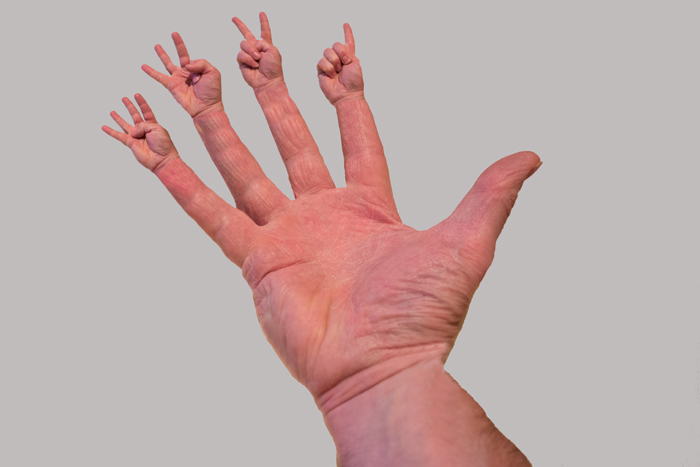This is a digitally altered photograph of a right hand, which is pale and Caucasian, with the palm facing out and the fingers outstretched towards the left corner. The background is a simple white-gray color, making the details of the hand stand out prominently. At the tips of each finger, there is a smaller hand. The pinky finger has a small hand with the thumb folded over, showing four fingers up. The ring finger has a small hand on it with the thumb holding down the index finger, revealing three fingers up. The middle finger's small hand has the thumb holding down the ring and pinky fingers, leaving two fingers up. Finally, the index finger has a small hand with only one finger up, as the thumb holds down the other three fingers. The veins in the wrist are visible, and while the small hands' fingernails are clear, the fingernails of the larger original hand are not visible. The image is evidently a piece of artistic work, showcasing an intricate countdown concept through the detailed manipulation of hands and fingers.